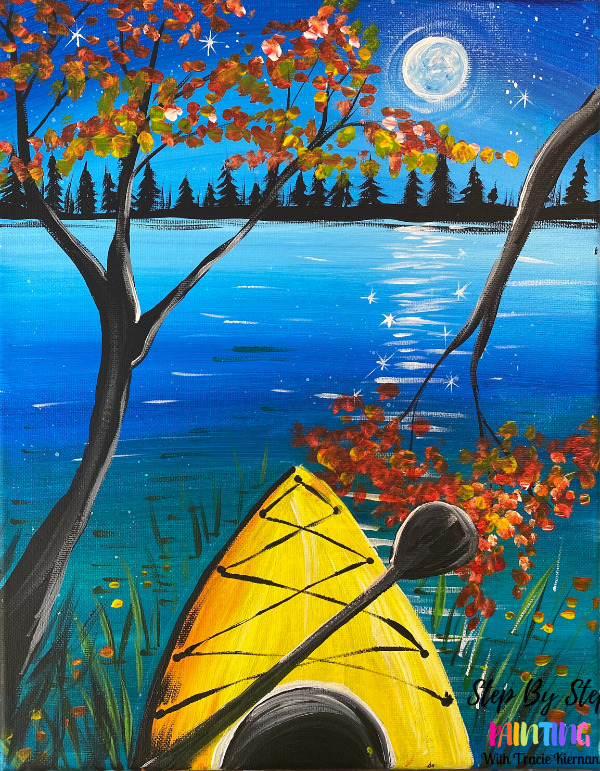This painting by Step by Step Paintings with Tracy Kiernan captures a tranquil night scene from the perspective of someone seated in a yellow kayak. The kayak, equipped with a black paddle resting on its bow, faces an expansive, serene lake that occupies the majority of the picture. The water softly reflects the moonlight from a bluish and white-gray moon high in the sky, casting a shimmering path across the lake's surface. The night sky is painted in deep, dark blue shades, subtly transitioning into lighter blue hues closer to the horizon. 

In the foreground, two trees with dark brown trunks and branches reach into the scene from either side of the kayak. Adorned with leaves in shades of green, yellow, gold, and orange, the trees frame the view elegantly, adding a touch of autumnal warmth. Scattered around the kayak in the water are delicate strands of seaweed or grass, enhancing the scene's natural feel.

Along the distant shoreline, a silhouette of shadowy evergreen trees stretches horizontally, creating a stark contrast against the illuminated sky. Above the treeline, a few sparkling stars accompany the moon, completing this peaceful nocturnal landscape. The painting is signed in the bottom right corner by the artist.